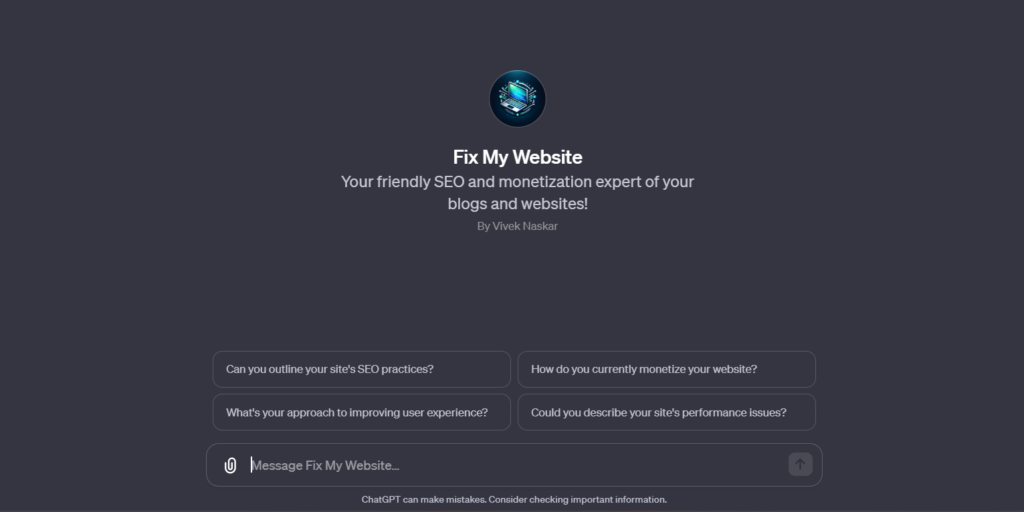Caption: 

The image depicts the homepage of a computer website titled "FixMyWebsite." The top and center sections of the page feature a gray background. Central to the design is a black circle containing an image of an open laptop, showcasing a blue screen and a gray casing. 

Beneath this graphic is a detailed text section. The first line, in large white letters, reads "FixMyWebsite." The following lines introduce the service with, "Your friendly SEO and monetization expert for your blogs and websites by Vivek Naskar." Vivek's name is spelled out for clarity: V-I-V-E-K N-A-S-K-A-R.

Below this introductory text, there are several outlined boxes positioned centrally, each containing specific questions to guide the user. These questions read:
1. Can you outline your site's SEO practices?
2. How do you currently monetize your website?
3. What's your approach to improving user experience?
4. Could you describe your site's performance issues?

At the bottom of these boxes, there is another line of text that states, "FixMessage, FixMyWebsite..." Further down is an advisory note in white font, warning users: "ChatGPT can make mistakes; consider checking important information."